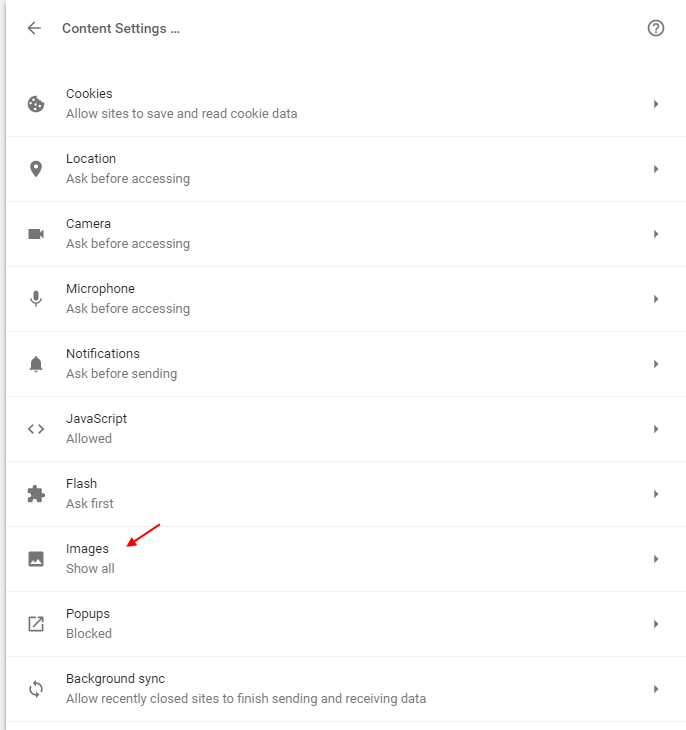This image is a screenshot of a web page, likely captured on a smartphone, characterized by a white background with all text displayed in gray font. At the top left of the page, "Content settings" is written in gray, alongside a left-pointing gray arrow indicating a return to the previous menu.

The page primarily consists of a vertical list of configurable settings:

1. **Cookies**: This section reads "Allow sites to save and read cookie data" with a right-pointing gray triangle indicating a drop-down menu option.
2. **Location**: Labeled with an inverted teardrop icon, it states "Ask before accessing."
3. **Camera**: Represented by a camera icon, it reads "Ask before accessing."
4. **Microphone**: Depicted by a microphone icon, it also states "Ask before accessing."
5. **Notifications**: Symbolized by a gray bell icon, it says "Ask before sending."
6. **JavaScript**: It states "Allowed" with a double-headed arrow indicating options or settings adjustments available.
7. **Flash**: Here, a gray splotch icon represents it, and it reads "Ask first."
8. **Images**: This section reads "Show all," and a red diagonal arrow points to this setting from the upper left.
9. **Pop-ups**: Marked as "Blocked."
10. **Background sync**: It states, "Allow recently closed sites to finish sending and receiving data."

The detailed layout and descriptions suggest this page allows users to manage various content settings, providing control over privacy and data usage features on their device.